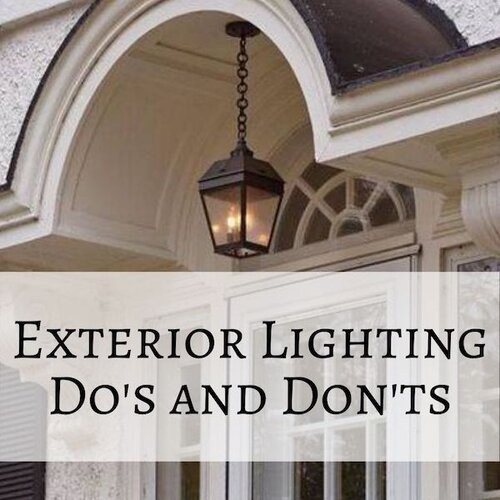In this detailed close-up image, an advertisement is prominently displayed with the bold black caption "EXTERIOR LIGHTING DO'S AND DON'TS" over a translucent white bar along the bottom. The focal point of the image is a well-lit, rustic brown lantern-style lighting fixture, hanging from a long black chain beneath an arched entryway ceiling. This archway, with its intricate molding and semi-circle glass window framed in white, sits above a door featuring at least six glass panels. The house itself has a classic, possibly colonial architecture, with beige and white exteriors, and a distinctive porch area. Subtle details like the light stains on the archway and the house’s beige trim add depth to the scene.